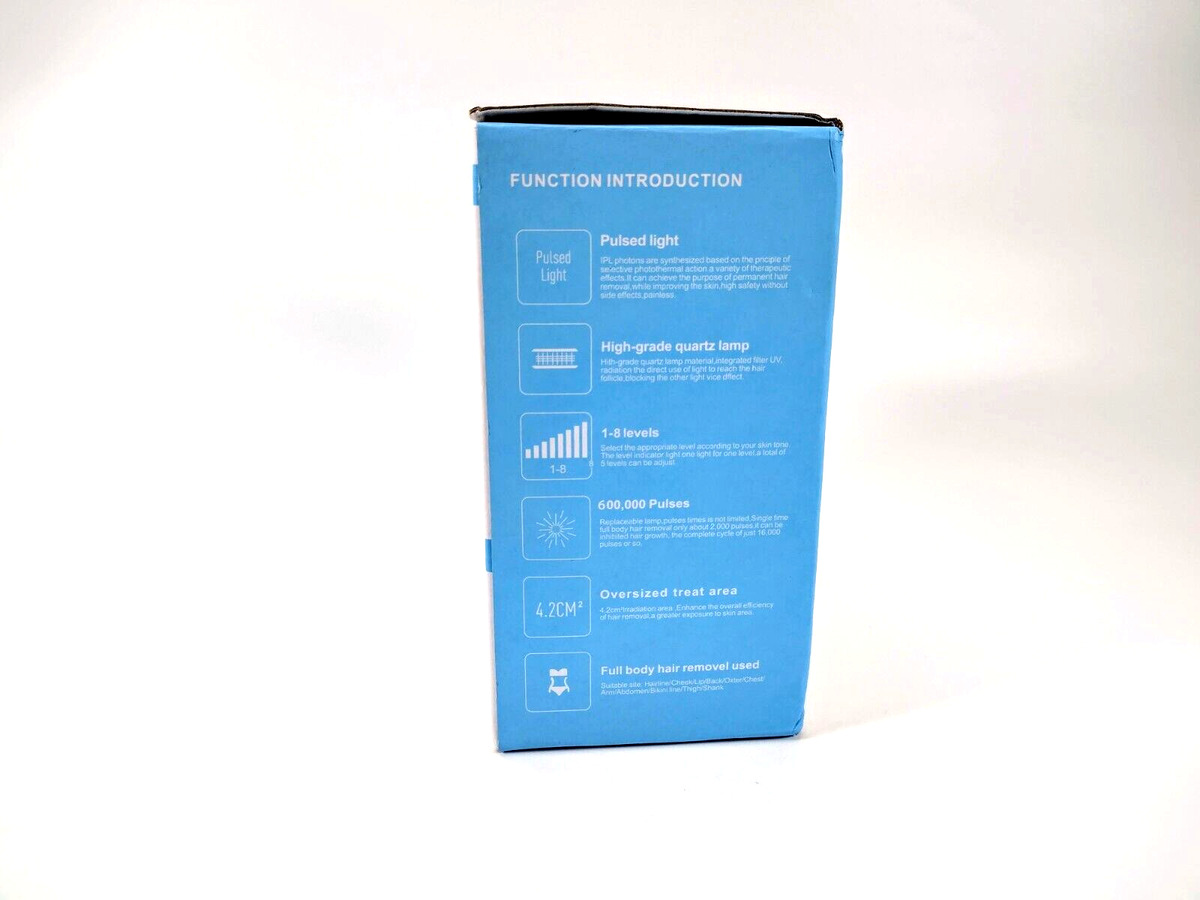This color photograph features a rectangular, sky-blue box with white text and graphics. The box is set against a well-lit, predominantly white background, with some grey shading on the right side. The top of the box is labeled "Function Introduction" in white text. Beneath this, there is a white square containing the words "Pulsed Light," alongside a block of text that is too small to read. Adjacent to this, an icon resembling the side view of a burger, depicting two solid parallel lines with a grid pattern in between, is positioned next to the label "High-Grade Quartz Lamp," followed by additional small text. Further down, an icon that appears to represent increasing bar levels is labeled "1 to 8 levels." Another graphic, shaped like a snowflake, indicates "600,000 pulses." A square on the left features "4.2 cm²," described as an "Oversized Treat Area." Lastly, an icon of a bikini at the bottom denotes the feature "Full Body Hair Removal Used." The box's design suggests it can open and close, emphasizing its practical and user-friendly packaging.